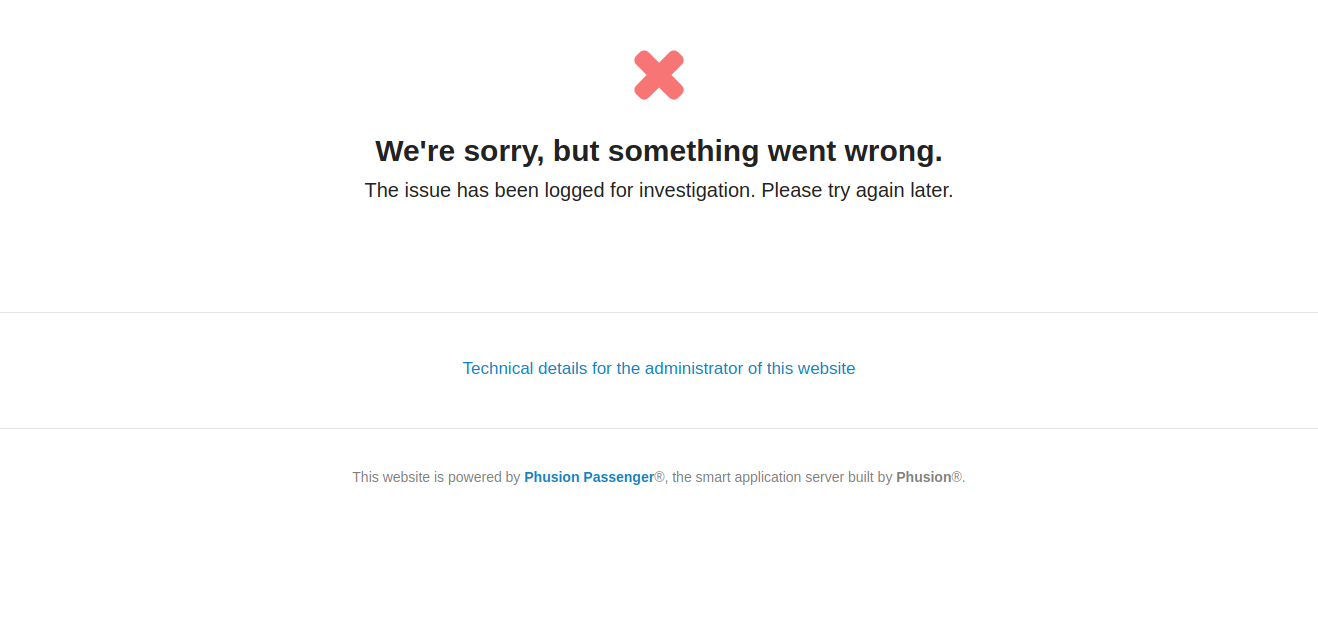This is a digital image taken from a website, displaying an error message. At the top of the image, there is a small red "X" icon. Directly below the icon, a bold, black-font sentence reads, "We're sorry, but something went wrong." Beneath this sentence, in a smaller black font, the text states, "The issue has been logged for investigation. Please try again later." A horizontal line separates this section from the next. Below the line, in blue font, which appears to be a hyperlink, the message states, "Technical details for the administrator of this website." Another horizontal line follows. Beneath this final line, also in blue clickable font, the text reads, "This website is powered by Phusion Passenger. The smart application server built by Phusion."